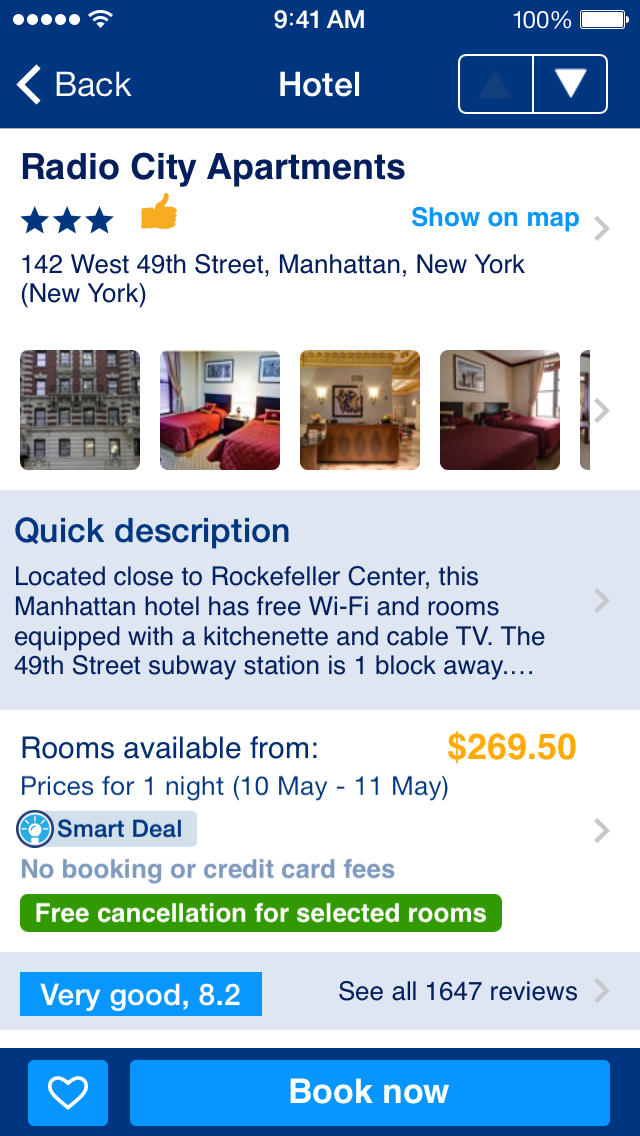This image depicts a device screen displaying information about a hotel. 

In the top-left corner, there are five white signal circles followed by a Wi-Fi icon. Centered at the top, the time is displayed as 9:41 AM. On the top-right, the battery status shows 100% with a battery icon next to it.

Below the top status bar, there is a navigation section. On the left, an arrow pointing left accompanies the word "Back." In the center of this section, the word "Hotel" is displayed. On the right, there are two square boxes; the left box is empty, while the right box contains a white, upside-down triangle.

Further down, the text "Radio City Apartments" is prominently displayed, followed by three blue stars and a yellow thumbs-up icon. The address "142 West 49th Street, Manhattan, New York (NY)" appears beneath the rating.

At the bottom of the image, there are four smaller images displayed horizontally. The first image on the left shows the exterior of the building, while the second image to the right depicts a room with two red beds.